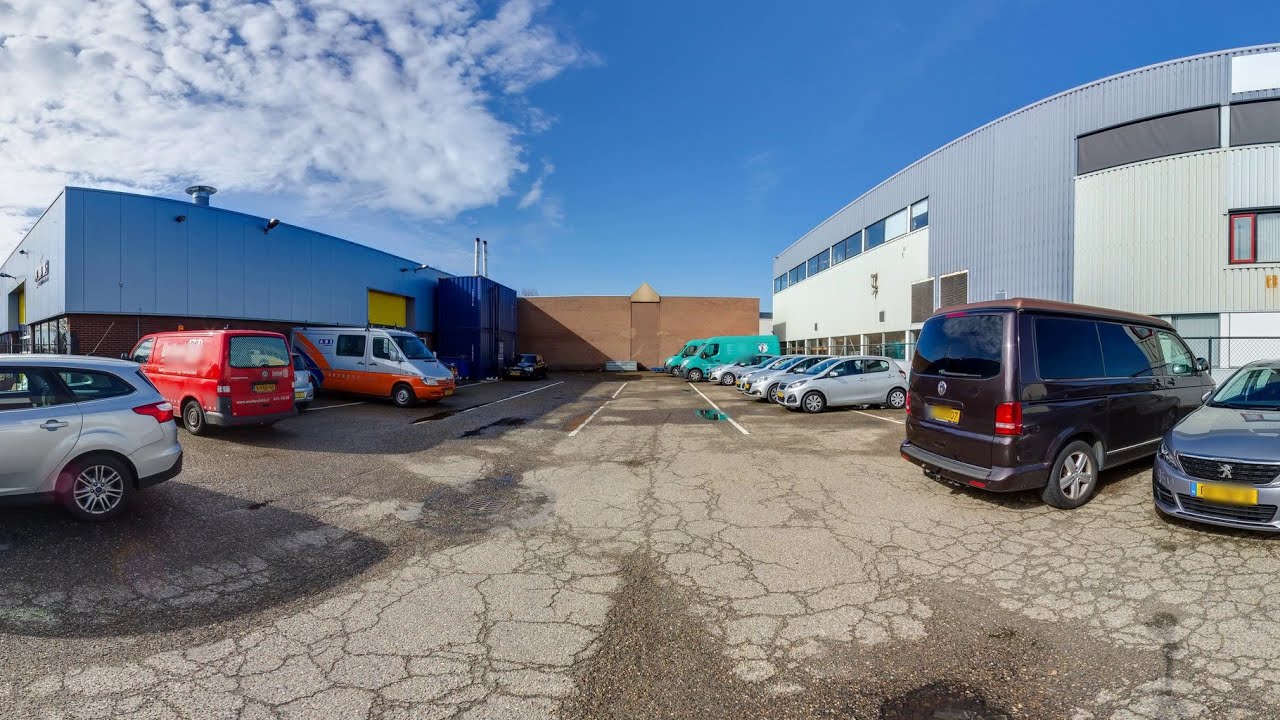The image captures a detailed scene of a weathered parking lot situated between three buildings forming a U-shape. On the right, there is a gray building, while straight ahead stands an orangish-brown building, and to the left, a bluish building with a yellow garage door. The concrete pavement appears old with numerous cracks and potholes, marked with white stripes indicating parking spaces. 

Several vehicles populate the lot, including a gray and orange van, a red van, and a partially visible silver sedan on the left. In the shadow of the central building, a car is partially obscured. On the far right of the lot are two turquoise vans and around four or five silver four-door vehicles. The foreground features a dark-colored van and another silver automobile. 

The sky is notably vivid blue with few clouds, offering a bright daytime ambiance despite the absence of direct sunlight in the picture. Contrasting sky details reveal white, cottony clouds on the left and a mostly clear blue expanse on the right, with only a hint of wispy clouds. The setting, likely a commercial area, is devoid of people and presents a panorama style blending two perspectives of the same site. The photograph emphasizes the rough condition of the pavement and the assortment of parked vehicles, indicative of a potentially bustling but currently quiet urban environment.